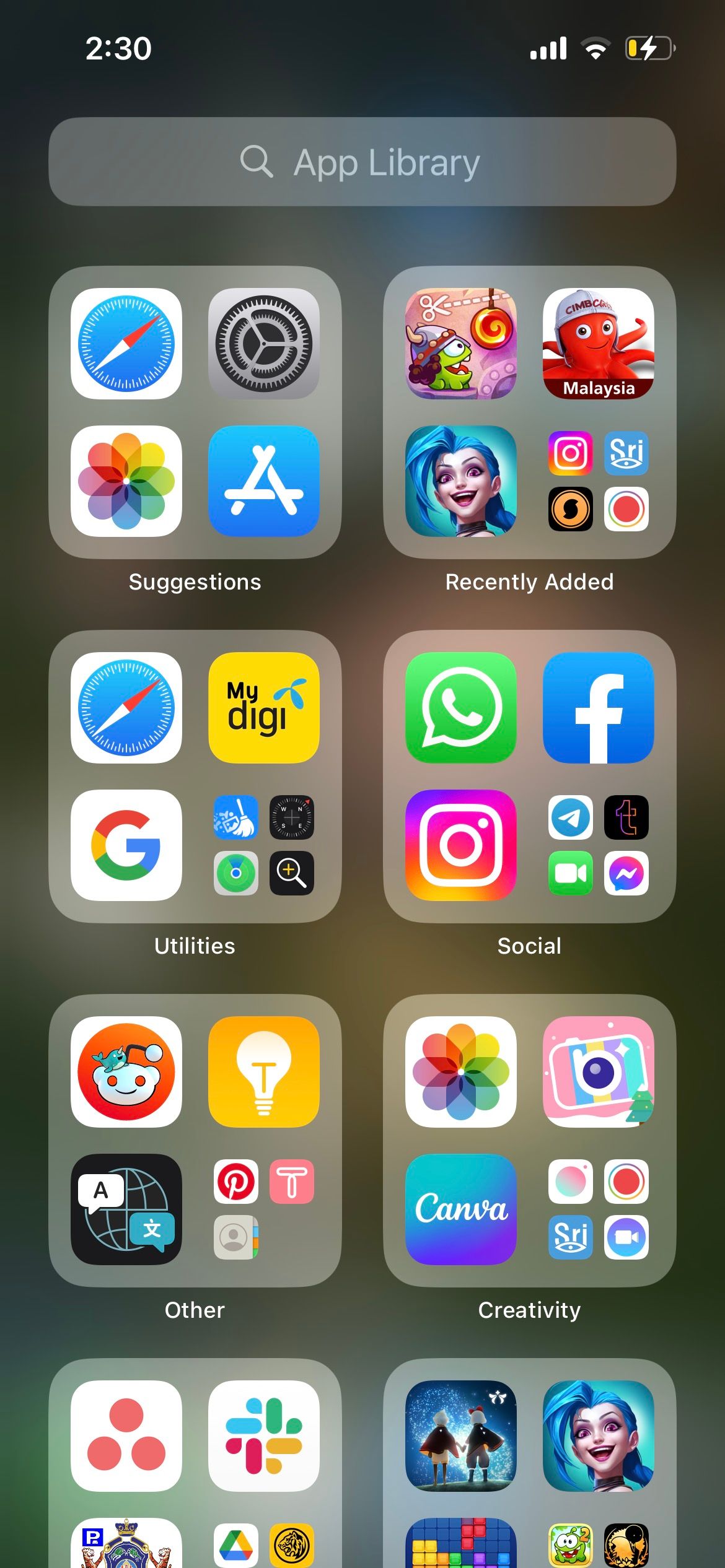In this image, a device displays its app library against a slightly blurry background. The app library header is visible at the top of the screen, with the time showing 2:30. The notification bar displays icons for Wi-Fi, a notepad application, and a charging battery.

Below the search bar, which reads "App Library," there are eight distinct folders organized into a grid. The first folder, situated at the top left, is labeled "Suggestions" and contains icons for Safari, Settings, Photos, and Browser. Adjacent to it on the right is the "Recently Added" folder, featuring three newly installed games and the Instagram app.

The third folder, "Utilities," houses apps such as Safari, MyDigi, Google, Calculator, Find My iPhone, Magnifier, and Clean. Below it, the "Social" folder includes WhatsApp, Facebook, Instagram, Telegram, Twitter, a video app, and Messaging.

The fifth folder, titled "Other," contains Reddit, Ideas, Pinterest, and additional icons. The "Creativity" folder appears next, with apps like Photos, Canva, and Record among others. The remaining two folders' names are not visible, but they are populated with various games.